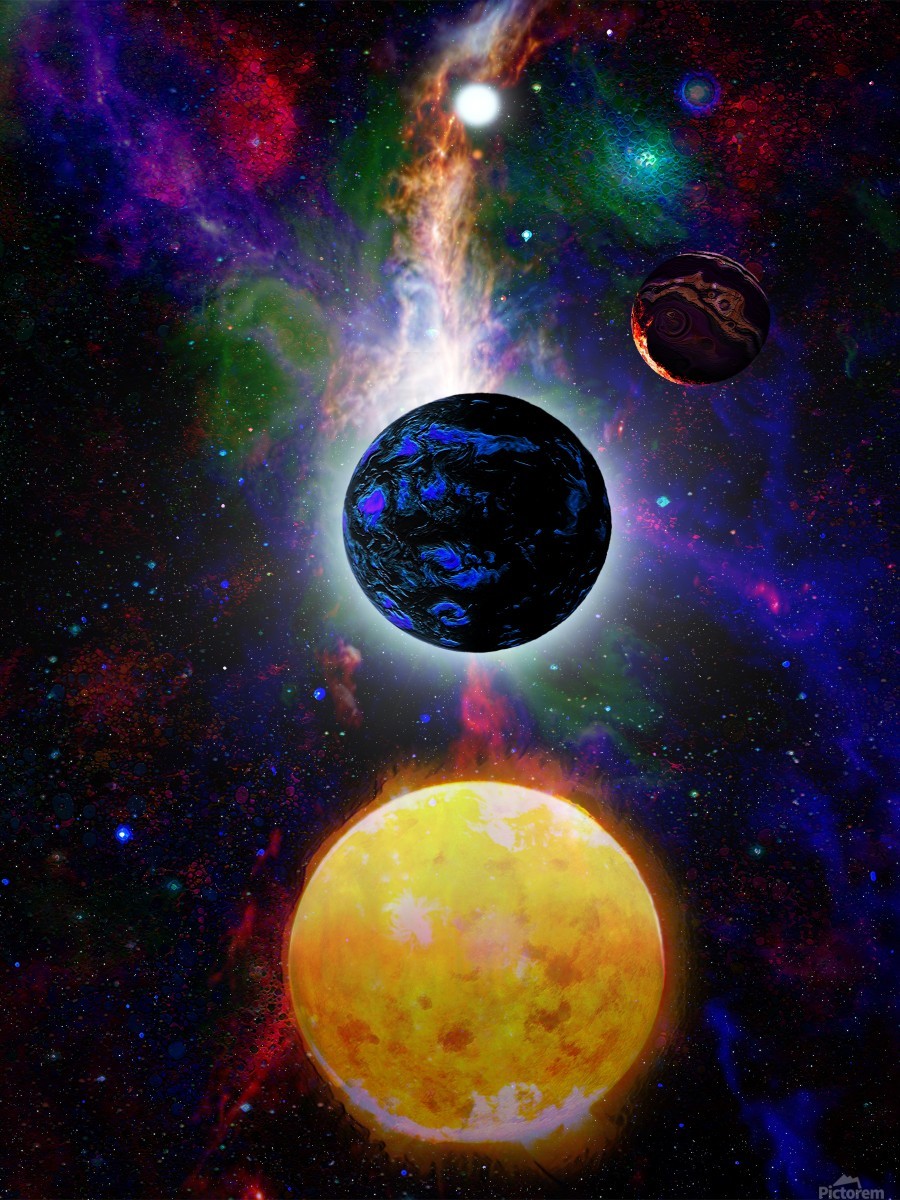This striking digital art piece vividly portrays a science fiction-inspired outer space scene. Dominating the lower center foreground is a vibrant yellow and red planet, possibly a sun, that radiates a glowing halo of orangish-yellow light. Behind this luminous orb is a smaller blue and black planet, enveloped in a white light halo that extends outward. In the distant right background is a large gas giant with a unique mix of dark purple, black, and tan, featuring swirling clouds and a distinctive tan strip with a black line running through it, reminiscent of a river.

The backdrop is a mesmerizing, dark expanse of deep space, accentuated by a colorful nebula exhibiting rich hues of red, green, purple, and blue. Scattered across this celestial canvas are bright spots representing stars, including a prominent white star. The entire composition conveys a sense of depth and spatial arrangement with the planets aligned but not to scale, adding to the surreal and otherworldly atmosphere. The image's meticulously crafted details, from the vividly colored gases to the cosmic glow, capture the essence of an otherworldly universe. The bottom right corner of the image features the text "pictorim".